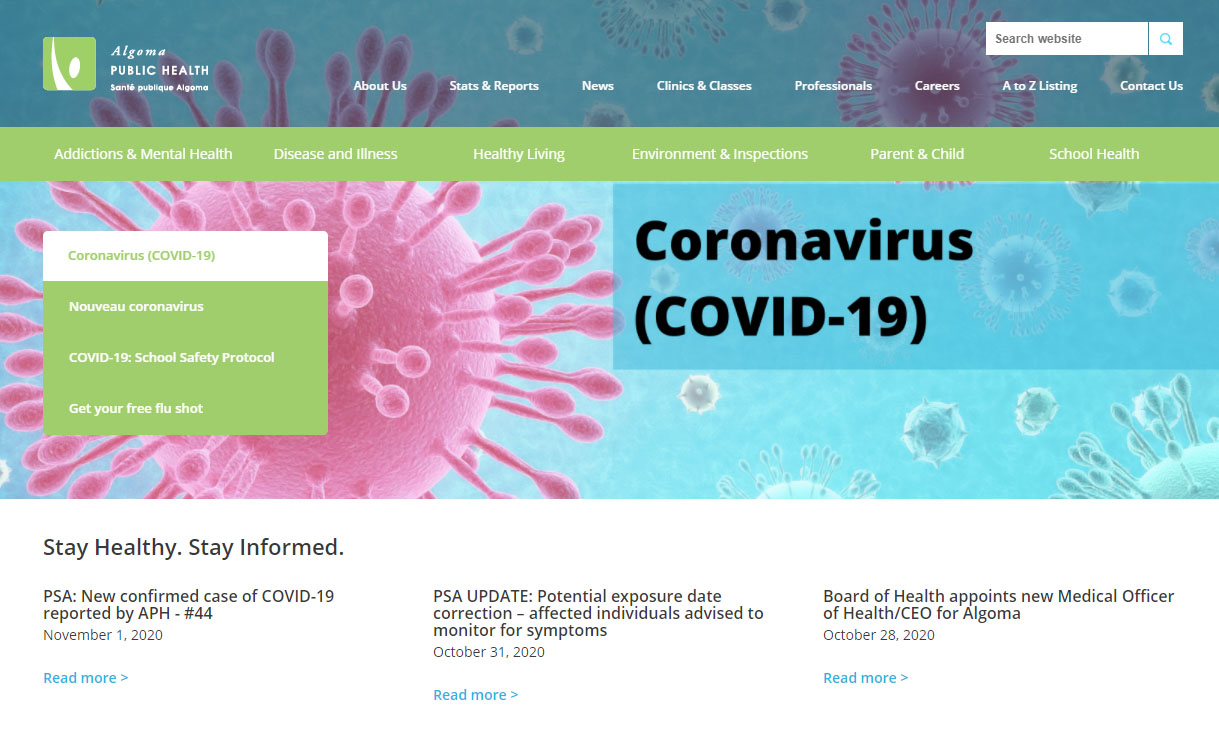The webpage displayed is from Algoma Public Health, featuring bilingual headings with "Algoma Public Health" and "Santé Publique Algoma" at the top. A small green icon of a person raising their hand is positioned alongside. To the right, there's a navigation menu with the options: "About Us," "Stats and Reports," "News," "Clinics and Classes," "Professionals," "Careers," "A-Z Listing," and "Contact Us," with a "Search Website" box displayed above.

The page includes green section tabs labeled: "Addictions and Mental Health," "Disease and Illness," "Healthy Living," "Environment and Inspections," "Parent and Child," and "School Health." Beneath these tabs, the word "Coronavirus" appears in black text, followed by "COVID-19" in parentheses. On the left side, there are several headlines: "Coronavirus, COVID-19," "NOVU," "Coronavirus, COVID-19, School Safety Protocol," and "Get Your Free Flu Shot."

The background features an illustrative blue design with red and blue virus icons, detailed with spike-like structures. Below this, text reads "Stay Healthy, Stay Informed," followed by a PSA noting, "New Confirmed Case of COVID-19 reported by APH-44." To the right, additional articles are listed with "Read More" links. One article is titled, "PSA Update, Potential Exposure Date Correction, Affected Individuals Advised to Monitor for Symptoms."